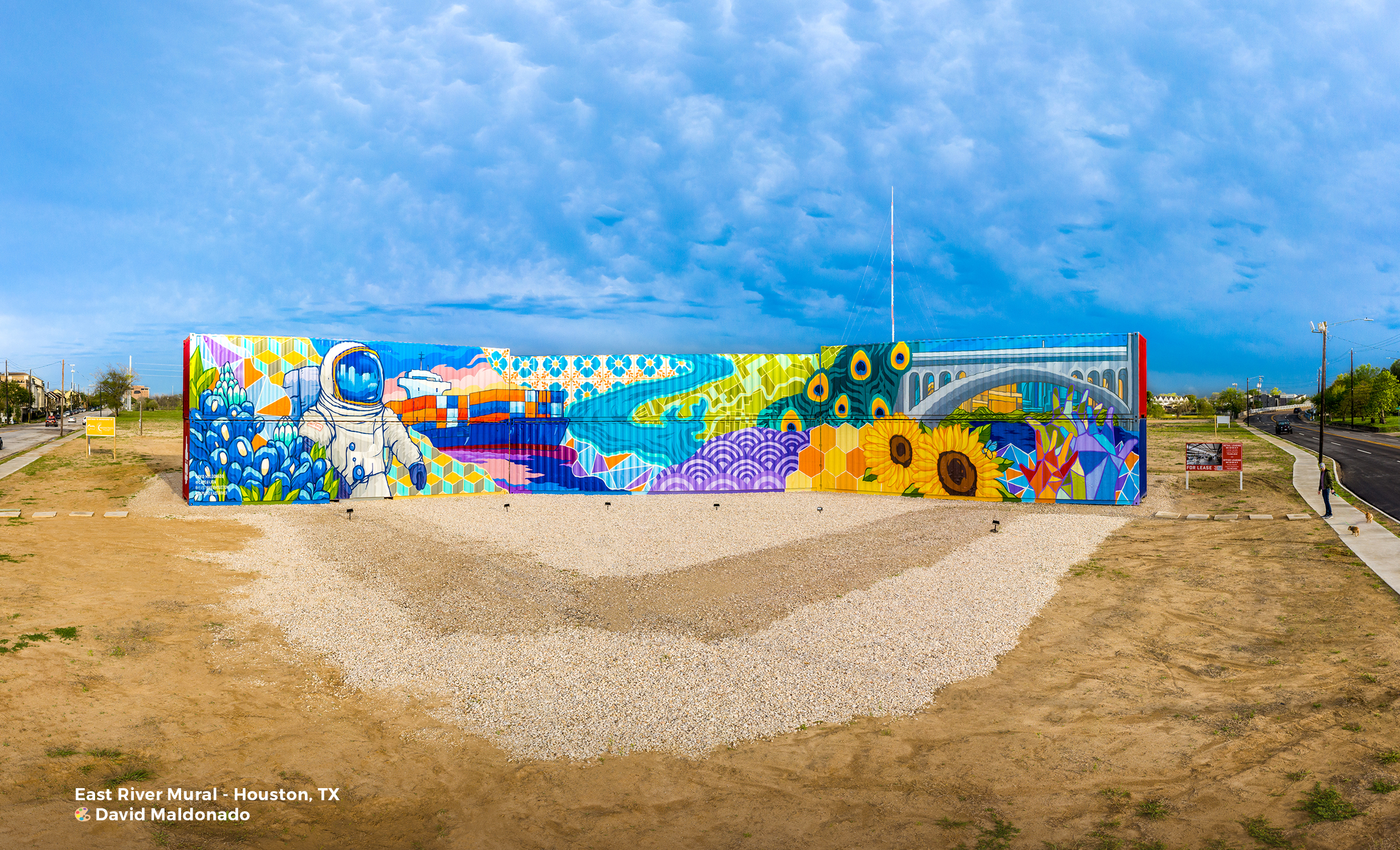This detailed landscape image, possibly an art piece, depicts the East River Mural in Houston, Texas, created by David Maldonado, as noted in the bottom left corner. The scene is set against a stunning blue sky filled with textured, wispy clouds that extend across the canvas. The ground below is barren, stretching out in shades of brown and tan, reminiscent of a desert landscape. 

Dominating the center of the image, the vibrant mural bursts with color and intricate designs. The top right features a gray bridge, while the left side showcases an astronaut in a white suit with a blue face covering. Surrounding the astronaut are vivid patterns, including sunflowers, bluebonnets, and various abstract shapes in lime green, yellow, and orange hues. Green and purple swirls, along with half circles, add to the mural's dynamic and lively appearance. 

In the mural's background, there are depictions of plants beneath the bridge, colored in blue, yellow, and green. The mural also includes a road and a sidewalk which runs alongside it, complete with a lamppost. The barren ground in front of the mural features light and dark sand curvatures, resembling rainbow arcs. Additionally, there is a sign adjacent to the mural indicating its significance. The surrounding area appears sparsely populated, contributing to the mural's prominence and the artwork's striking contrast against the desolate terrain.